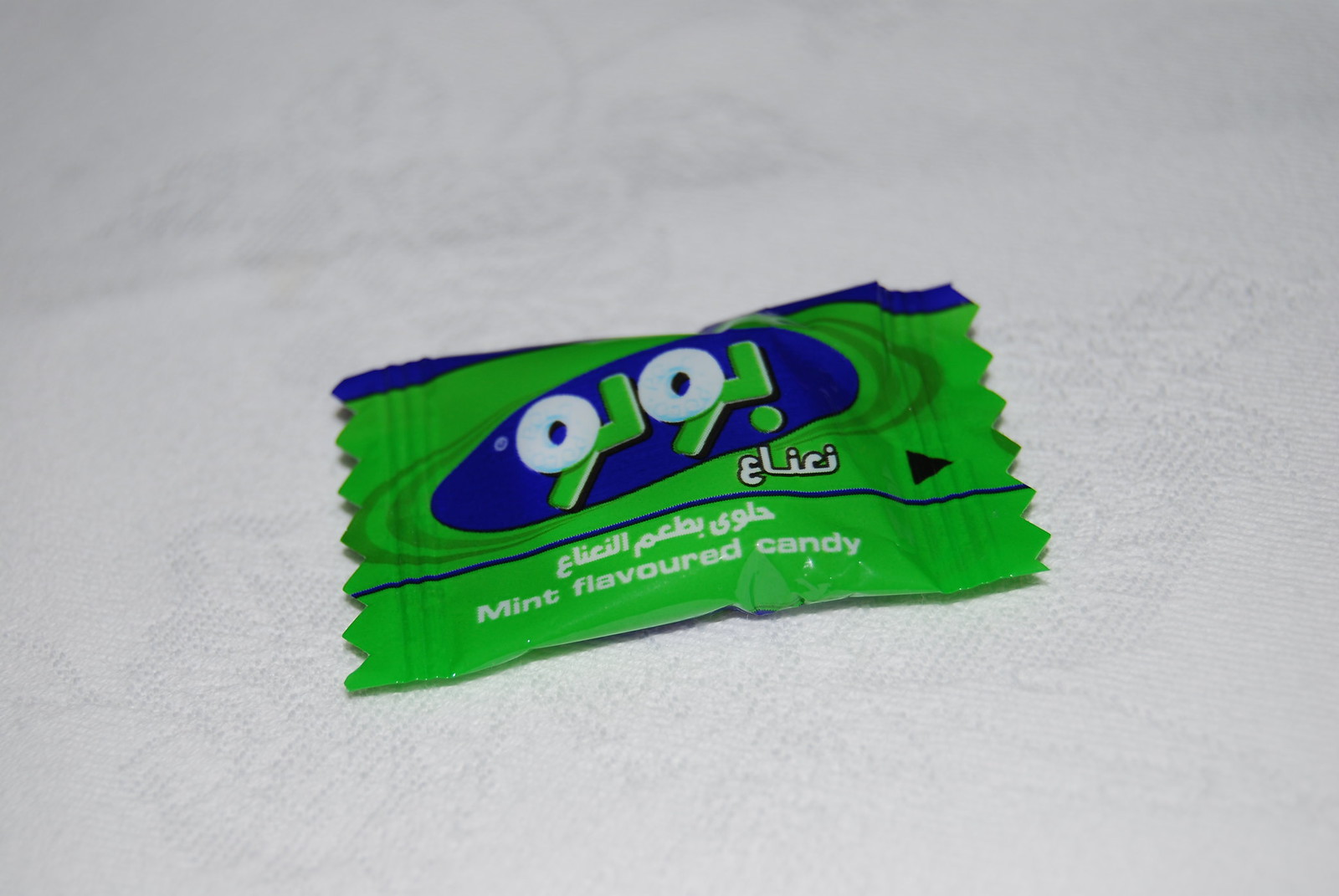A close-up photograph features a small piece of candy in a crumpled, plastic wrapper lying on an intricate, white embroidered cloth resembling a tablecloth or curtain, possibly with a floral pattern. The candy wrapper, predominantly bright green with blue accents, includes a blue circle or oblong shape surrounding a logo in the center. The logo consists of stylized characters resembling "O backwards L, O backwards L," where the O's appear like Polo mints. There is Arabic text beneath the logo and the phrase "mint flavored candy" written in white. The wrapper also contains a blue arrow indicating where to open the candy.